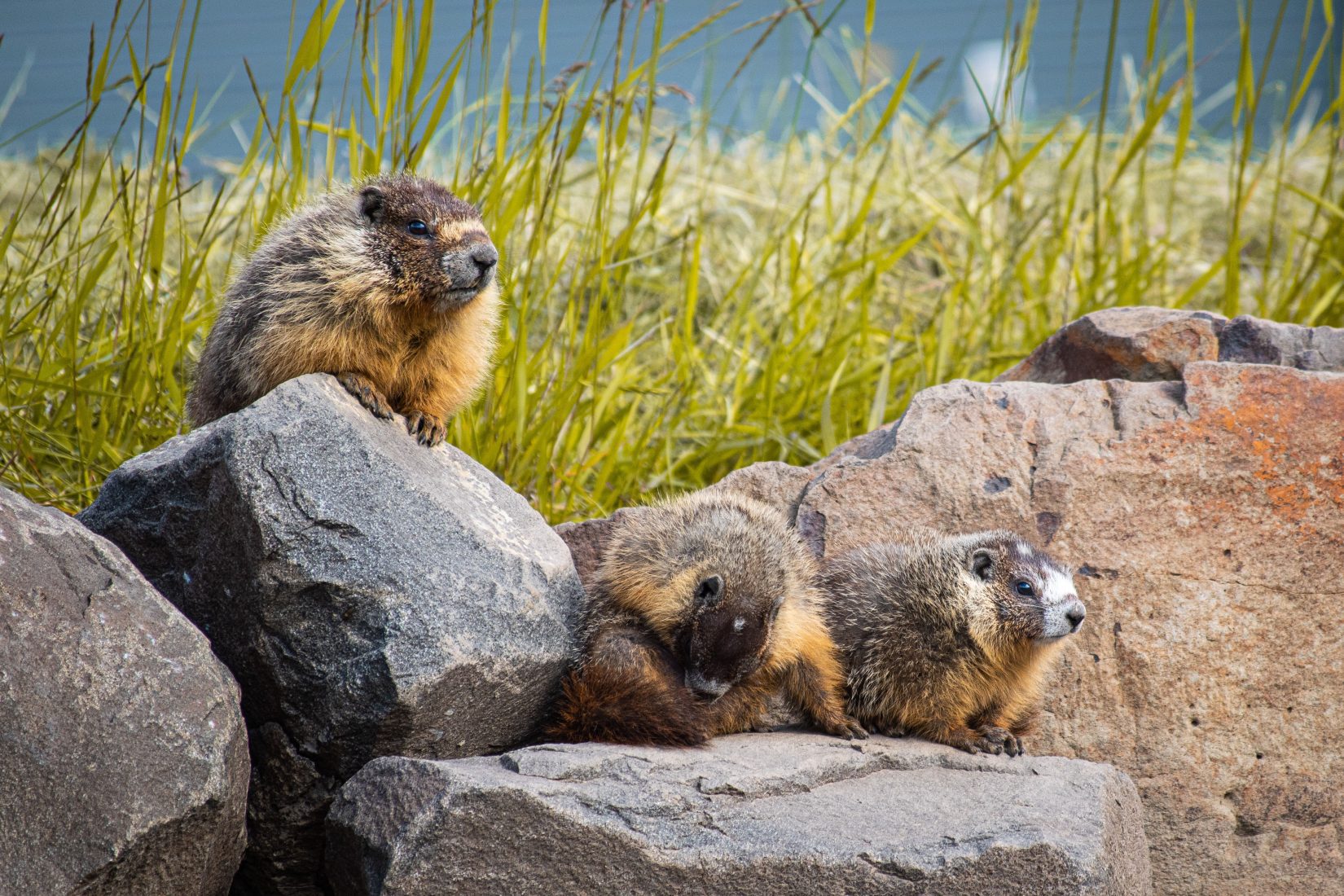In this landscape-oriented photograph, three fluffy rodents, possibly groundhogs or beavers, are prominently featured. The rodent on the left stands tallest, perched atop a large rock, while the other two rest on flatter, slightly lower rocks. All three have light brown chests, darker heads, and black eyes, with a distinctive preening behavior noted in the middle rodent, which is focused on its tail. Their placement is on a line of boulders, likely man-made, with tall green weeds and grass stretching into the background. In the distance, a vivid blue water body extends, suggesting a beach-like, swampy environment. The overall scene is bathed in sunlight, casting clear shadows and highlights on the rocks, enhancing this tranquil snapshot of nature.